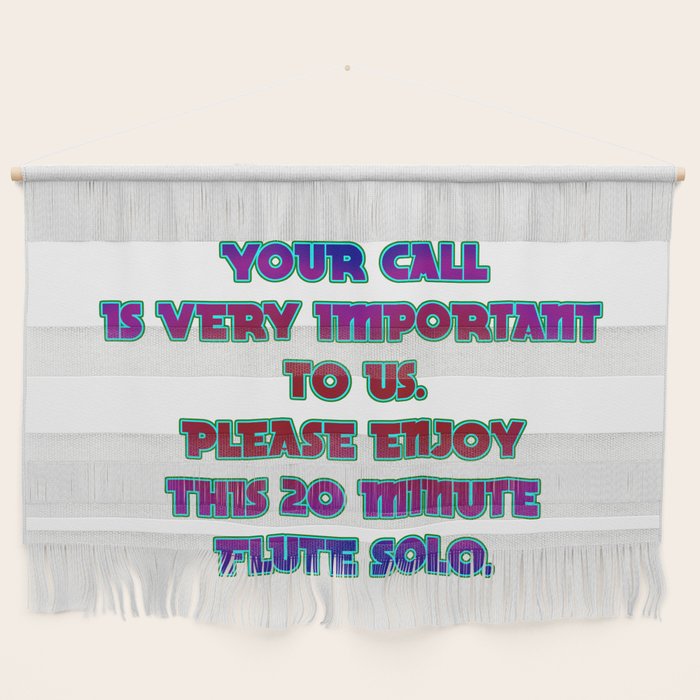This image showcases a charming and humorous wall tapestry. The tapestry features alternating gray and white stripes, with a thin white stripe near the bottom, ending in gray fringes. It's attached to a wall via a string and bar, which is pinned in place, possibly with a thumbtack. The backdrop is a white wall. Written across the fabric in a playful, futuristic serif font, is the phrase, "Your call is very important to us. Please enjoy this 20-minute flute solo." The lettering transitions in color throughout the text from purple at the top, to red in the middle, and back to purple towards the bottom. Comically, part of the phrase, particularly the 'flute solo,' is embedded within the fringes at the bottom, making the statement an amusing nod to customer service experiences.